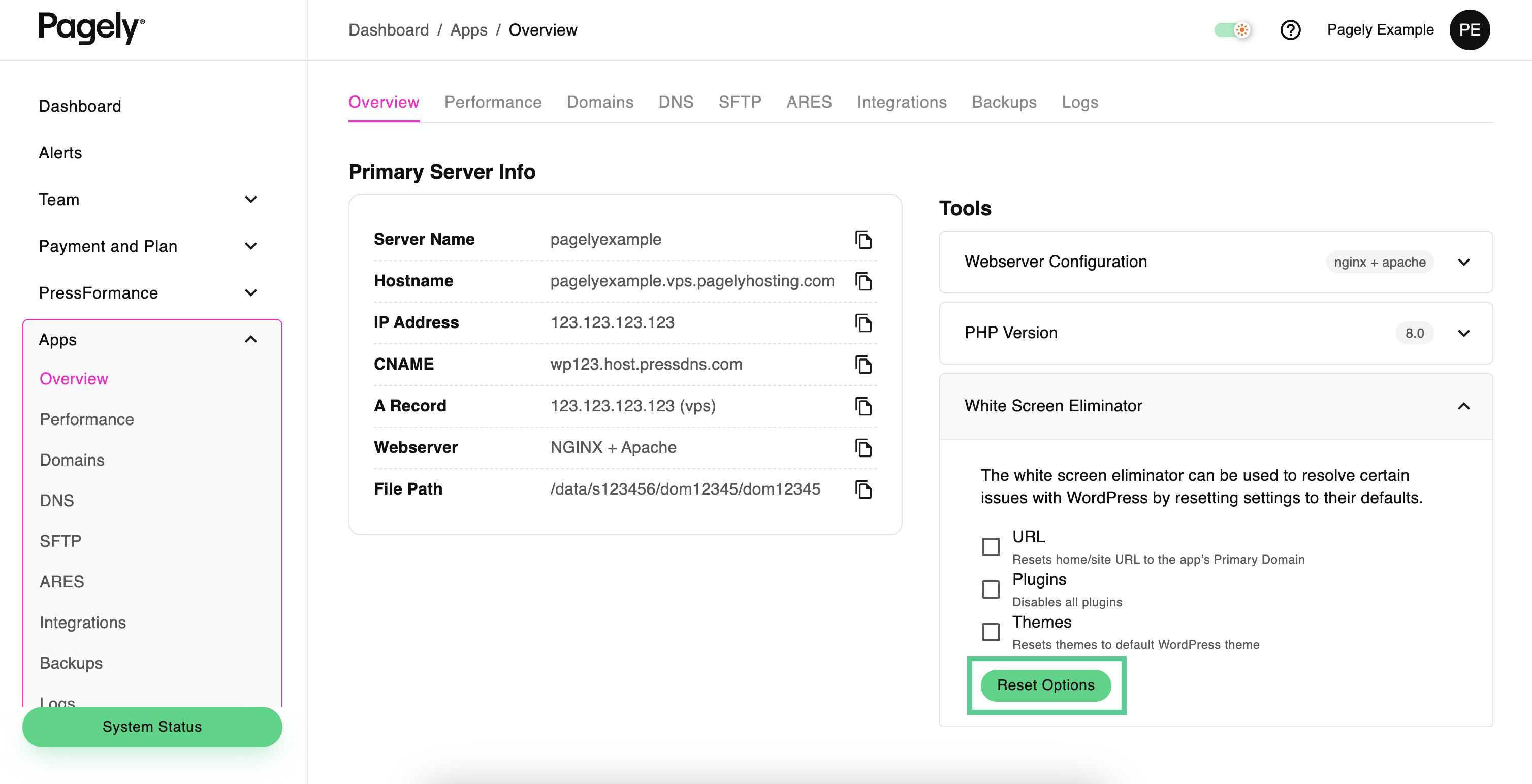This detailed image caption for a Pagely screenshot has been cleaned up for clarity and detail:

"This screenshot showcases the Pagely interface. The header in the upper left-hand corner prominently features the bold 'Pagely' logo. Adjacent to this logo is a concise menu with options labeled 'Dashboard,' 'Apps,' and 'Overview.'

On the left side of the image, a vertical sidebar presents a comprehensive navigation menu including: 'Dashboard,' 'Alerts,' 'Team,' 'Payment,' 'Plan,' 'Press Performance,' 'Apps,' 'Overview,' 'Performance,' 'Domains,' 'DNS,' 'SFTP,' 'ARES,' 'Integrations,' and 'Backups.'

The main content area begins with a horizontal strip menu in black text on a white background, with the selected text highlighted in purple. The options here mirror some of the sidebar items, listing: 'Overview,' 'Performance,' 'Domains,' 'DNS,' 'SFTP,' 'ARES,' 'Integrations,' 'Backups,' and 'Logs.' The page displayed below the menu strip focuses on the primary server information and tools, corresponding to these menu selections. As 'Overview' is selected at the top, it indicates the primary view is currently on the 'Overview' page."